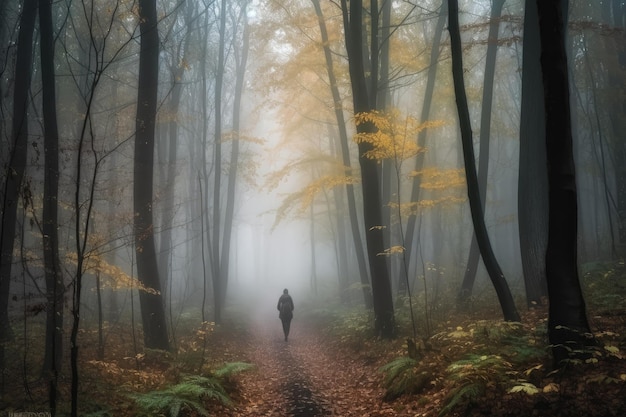In this slightly dark and misty forest, the air is thick with fog, casting an eerie and lonely atmosphere. Tall trees, their details obscured by shadows and mist, stretch upwards, forming a dense canopy of silhouettes that reach heights of 50 feet or more. A path strewn with fallen, orangey-yellow leaves runs through the center of the image, wide enough for a car, with grooves on either side and a raised, dark center. Walking down this path is the silhouette of a woman, heading away from the viewer. She wears a long coat, a backpack, and possibly a hat, her form blending into the blackness and fog that envelop her. The blanket of fog ahead deepens, with the path disappearing into the mist, as some trees retain their golden leaves, adding pockets of color to the otherwise gray and shadowy forest.